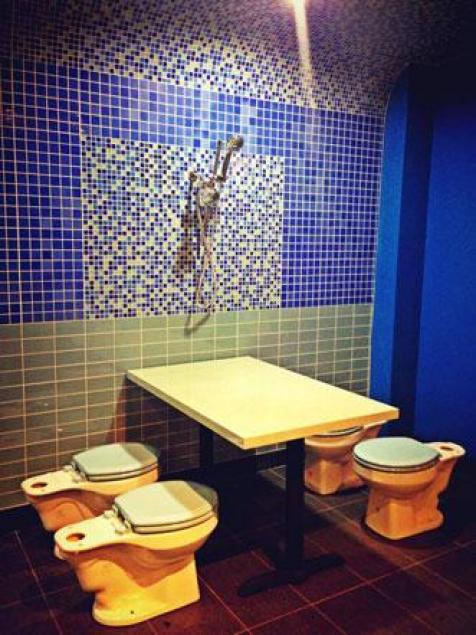The image portrays a bathroom-themed dining setup, suggesting an artistic installation rather than a functional space. The room features an eclectic mix of green, blue, and collage mosaic tiles, with a distinctive arching roofline. Dominating the center is a white table with black legs, but instead of conventional chairs, four closed-lid toilets are arranged around it, two on each side, facing each other. These toilets have large holes at the back, hinting at incomplete plumbing. A shower head with a detachable handle is mounted on the mosaic-tiled wall above a rectangle of gray tiles. The mosaic includes varied patterns: from green, rectangular tiles with tan caulking at the bottom to small blue and white squares surrounding the shower area, bordered by darker blue tiles. This unique setup, complete with a brown-tiled floor, likely serves as an art piece given the unconventional combination of dining and bathroom elements.